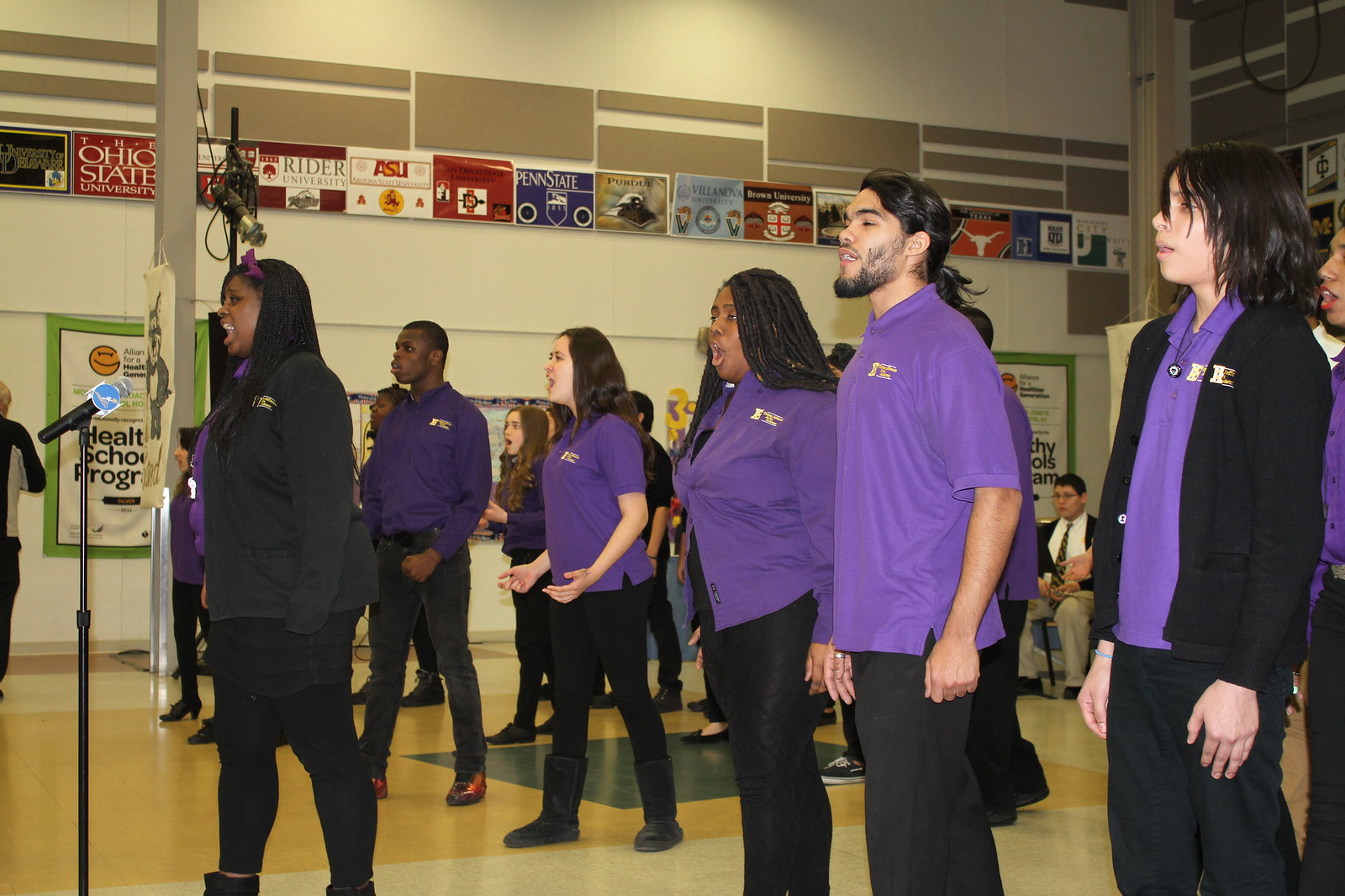The image depicts a color photograph of a diverse group of young adults, likely college-age or late teenagers, gathered in a gymnasium or large program space. The majority of the performers are dark-skinned, either Black or Hispanic, with a few White individuals. Most have black hair, except for a White girl with dark brown hair. At the front left, a Black girl with long dark hair, dressed in a black top, black skirt, and black leggings, stands in front of a microphone, possibly leading the performance. 

The performers, arranged in a double row, wear varying styles of the same purple shirts emblazoned with gold writing on the upper left chest. Some are also wearing black jackets. All are facing to the left, appearing to sing, with mouths open and heads held high. Behind them, the gym's white walls are adorned with colorful posters and signs from various educational organizations, including Ohio State University, ASU, and Penn State.

In the background, a person in a black suit jacket, colorful tie, and khaki pants sits in front of a music stand, holding a musical instrument, suggesting a combined singing and musical performance. The smooth gym floor and the sports section posters on the side enhance the backdrop, indicating this might be an event or convention showcasing sports schools.